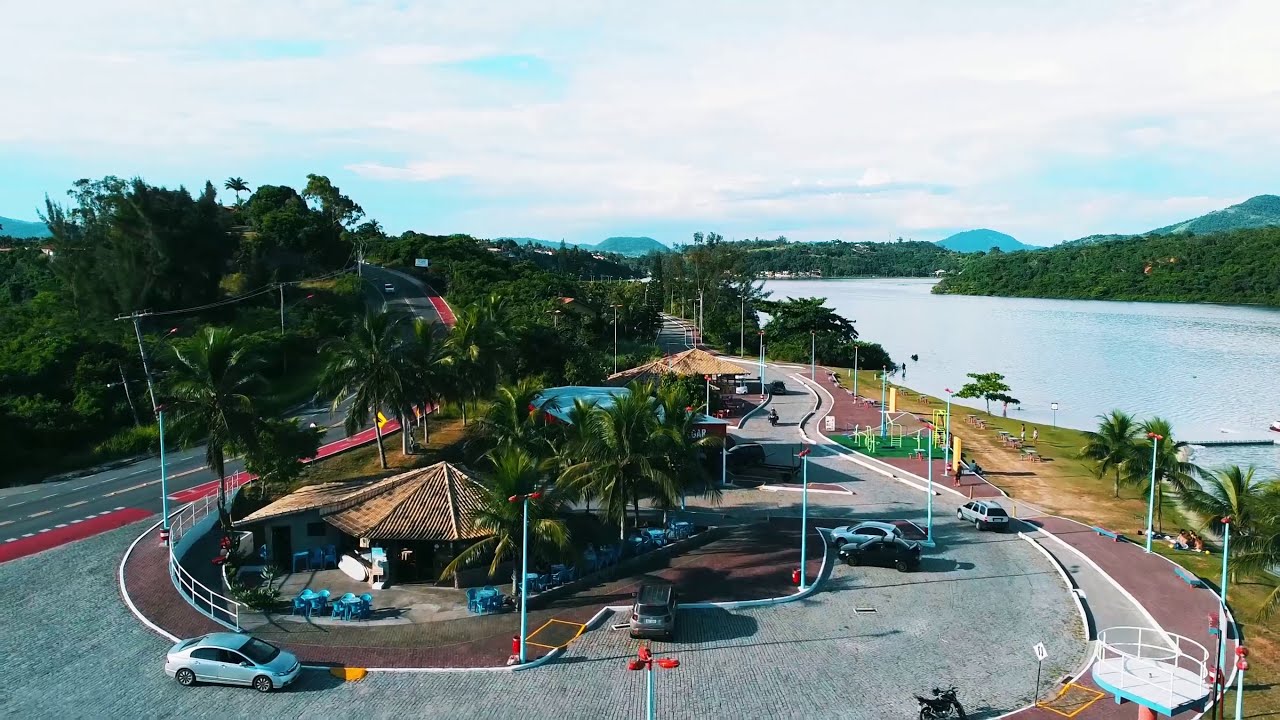This aerial image captures an outdoor parking area during the daytime, primarily focused on a central island-like area containing several structures with domed, hut-like, or octagonal roofs constructed of light tan tiling. These structures, potentially small restaurants or picnic spots, are surrounded by blue chairs and tables, and are dotted with tall, green palm trees. The parking lot itself forms a roundabout, encircling these central buildings. Off to the right-hand side of the image, a wide, winding river with shiny blue water flows next to a grassy and sandy embankment populated by small pine trees. Beyond the river, rolling hills with lush green terrain and some mountainous ranges can be seen in the distance. The left-hand side of the image showcases a traditional blacktop road bordered by more tall, green trees and foliage. The weather appears slightly hazy with a predominantly cloudy sky, allowing a few patches of blue to peek through.